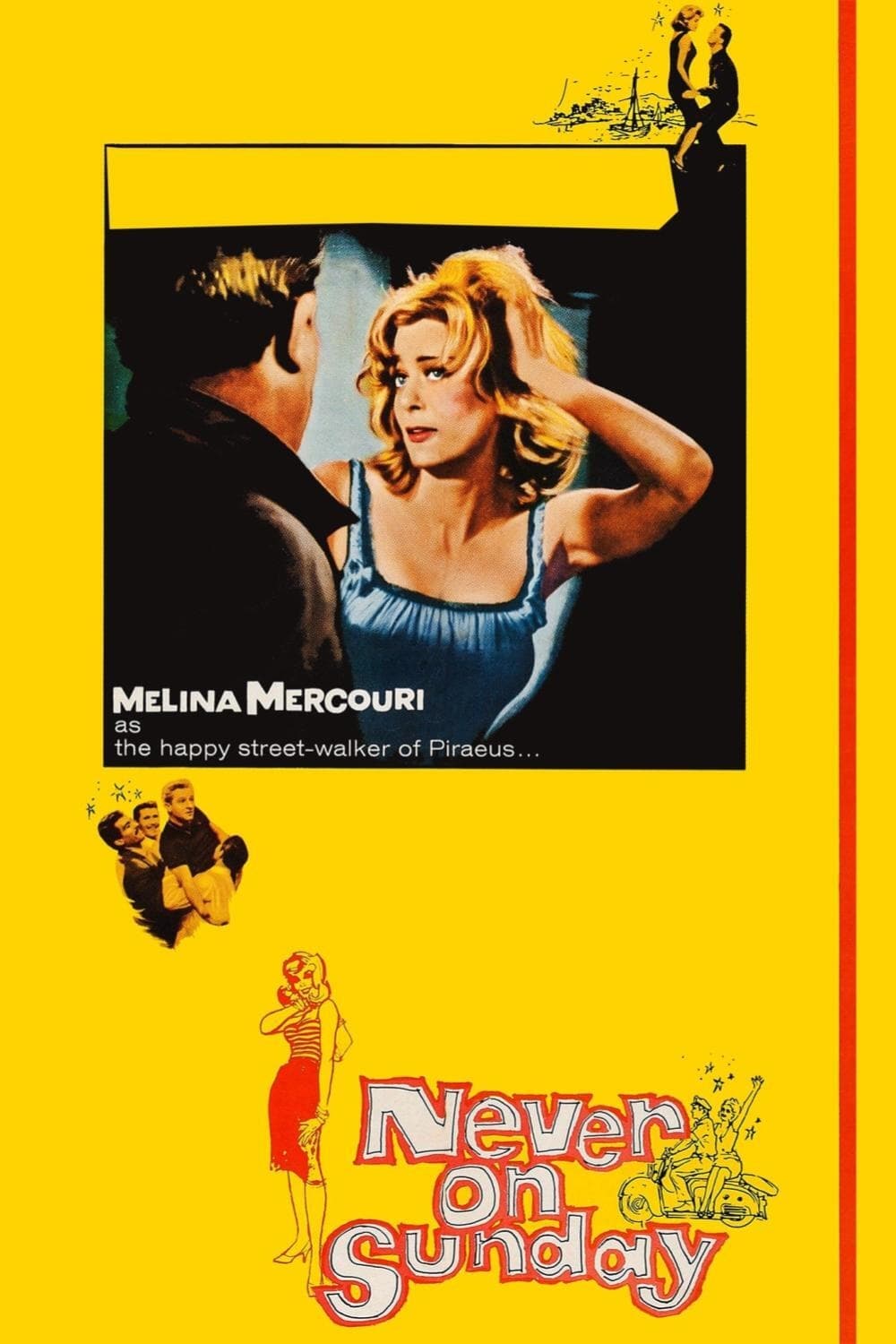This vibrant yellow poster, predominantly featuring a thin red stripe down its right-hand side, appears to advertise a film or theatrical production. Dominating the upper half of the poster is a photograph of a woman in a blue dress, with her hand in her hair, looking curiously or concernedly at a man with his back to the viewer. He wears a brown coat with a popped collar. The central square of the poster highlights the lead actress, Melina Mercouri, labeled as "the Happy Streetwalker of Piraeus." Illustrations include one with three men, where one holds either a child or a woman, and another of the couple dancing against a scenic mountain backdrop. At the bottom right, text reads "Never on Sunday," accompanied by two graphics: one of a woman in red and another blue one of a man and woman on a motorcycle. The overall design is styled with old 1900s caricature and lettering, evoking a vintage feel.